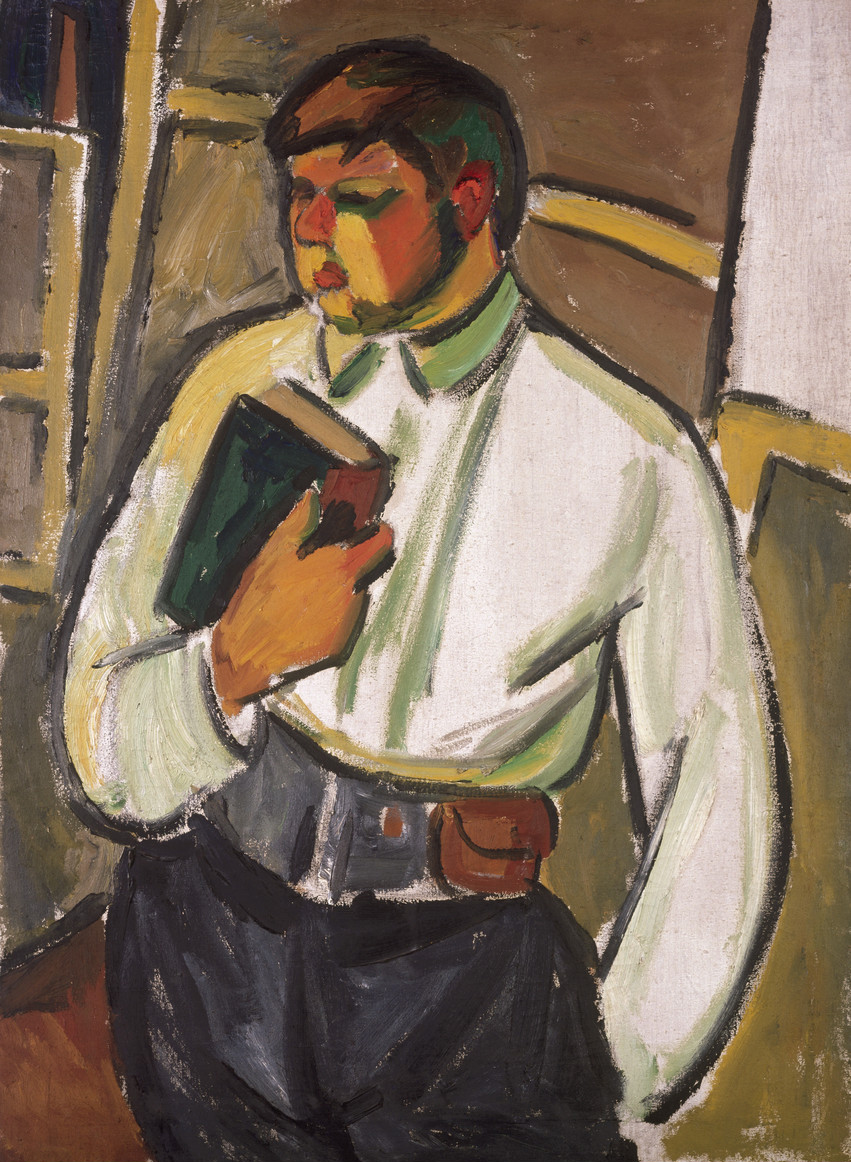This vertical rectangular painting depicts a man indoors, standing in front of what appears to be a brown brick wall. The man, looking slightly downward with pursed lips, has sparse brown hair on the top of his head and a mustache. His face is predominantly an orange hue, with a flesh-toned beige area contrasting it. He is dressed in a white, long-sleeved, button-up shirt with a green collar. His left hand is tucked into the pocket of his black pants, while his right hand holds a green hardbound book with a dark brown binder edge close to his chest. Around his waist, he wears a wide belt with a leather wallet attached to it. The background includes a brown structure, possibly a door, with an adjacent brown element that might be a window, and to the right, a gray wall with a painting frame. The color palette of the painting utilizes tones of white, black, green, brown, and touches of yellow.